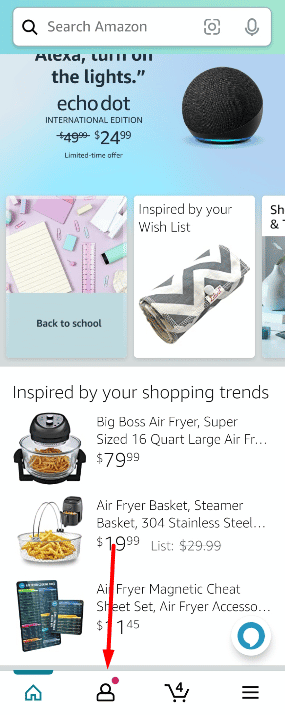Here is a refined and detailed caption for the given image:

---

This image showcases an Amazon e-commerce website displayed on a mobile device in portrait orientation. The top half of the interface features a light blue gradient, transitioning to light gray. Prominently positioned at the top is an aqua-colored bar with a white search bar overlay. Inside the search bar are the words "Search Amazon," a black magnifying glass icon, an icon resembling a dashed square with a circle (potentially for photo search), and a microphone icon for voice search.

Beneath the search bar, on the blue backdrop, is a photograph of a spherical black Echo Dot (referred to as 'charcoal'). Adjacent to the device is the quote, “Alexa, turn on the lights,” followed by text that reads "Echo Dot International Edition $49.99," with the price slashed out and updated to "$24.99." This is labeled as a "Limited time offer."

Below this, three shopping category tiles are presented, with the first two fully visible and the third partially cropped. The leftmost tile, captioned "Back to School," displays a photograph of organized school supplies such as rulers, paper clips, Post-it notes, and notepads against a purple background. The second tile, titled "Inspired by your Wish List," shows a soft eyeglass case with a gray and white zig-zag pattern on a white background. The third tile, only partially visible, seems to begin with "SH" and includes an ampersand below, alongside what appears to be part of a photo featuring a bud vase.

The bottom half of the screen highlights items under "Inspired by your shopping trends," displaying three products with images and descriptions aligned to the left. The first item is the "Big Boss Air Fryer," described as a "Super Sized 16 Quart Large Air Fryer" priced at $79.99. The second is an "Air Fryer Basket Steamer Basket, $3.04, Stainless Steel," listed at $19.99 but originally priced at $29.99. Finally, there's an "Air Fryer Magnetic Cheat Sheet, Air Fryer Accessory," which appears to be priced at $11.45, though the visibility is partially obstructed by a large red downward arrow. This arrow points towards the bottom of the screen, where an icon of a person with a red notification dot is located, indicating the account section.

Additionally, a blue circle to the right of the arrow contains a white speech bubble, likely representing the chat function. Along the bottom of the screen, four main navigation icons are visible: a home button, an account icon with a red dot, a shopping cart icon displaying the number four (indicating four items in the cart), and a triple-stack menu icon.

---